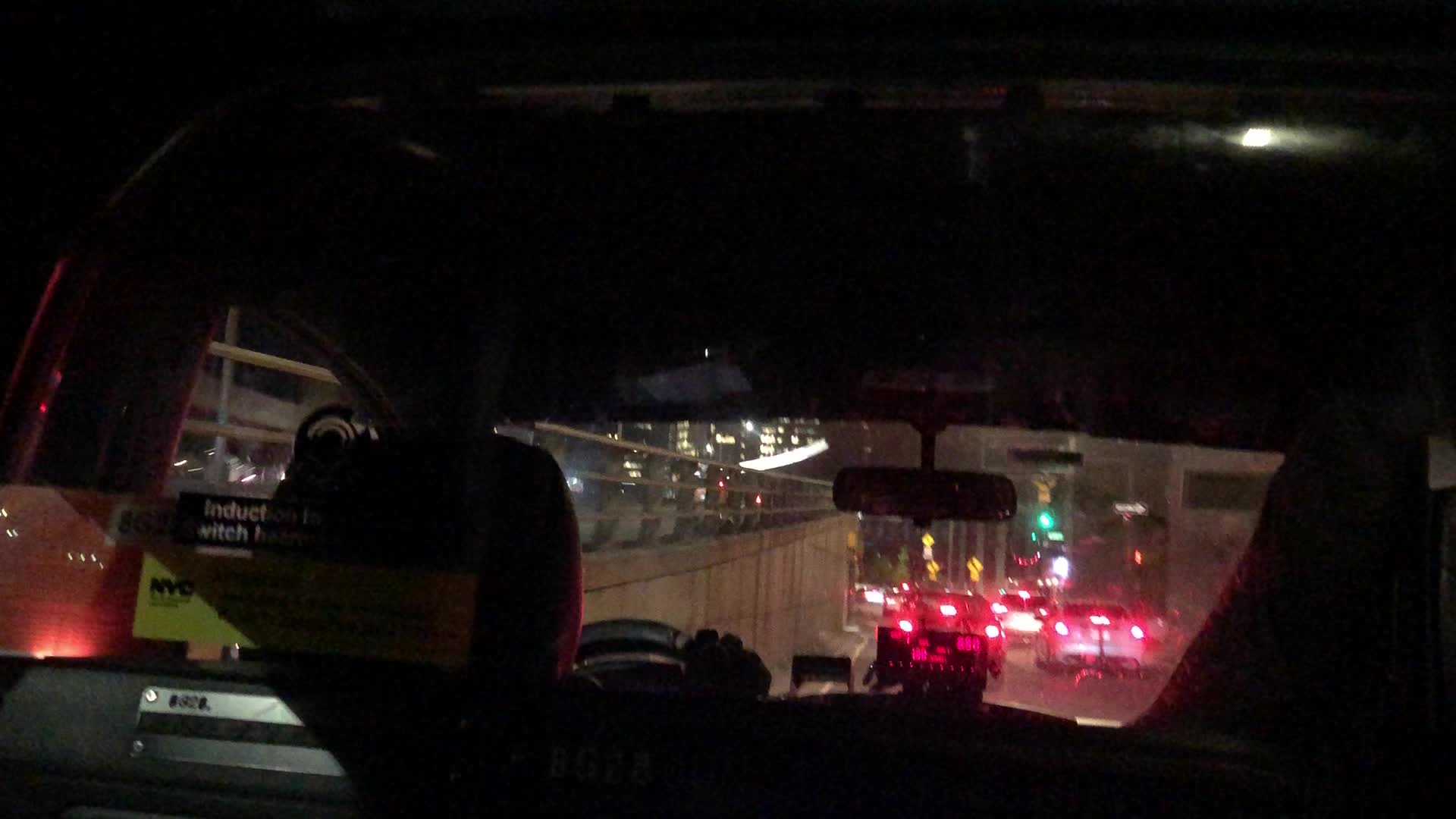This is a nighttime color photograph taken from the back seat of a darkened car, likely a taxi. The car is descending into an underpass or possibly navigating a freeway. Ahead, there is heavy, stopped traffic, evident from the numerous red taillights of the cars ahead in both lanes. The green traffic light in the distance indicates that it's probably just turned green or the vehicles haven't yet moved forward. The car's interior is dimly lit, with the driver's hand visible on the left-side steering wheel, suggesting this is likely in a country like the United States. To the left side of the image, a railing runs alongside a concrete wall, providing additional context that the car is moving adjacent to an industrial-looking infrastructure. Above the road, tall urban structures hint at a metropolitan setting. The rear of the driver's seat displays a sign with "NYD," reinforcing the possible location as being in or near a city.